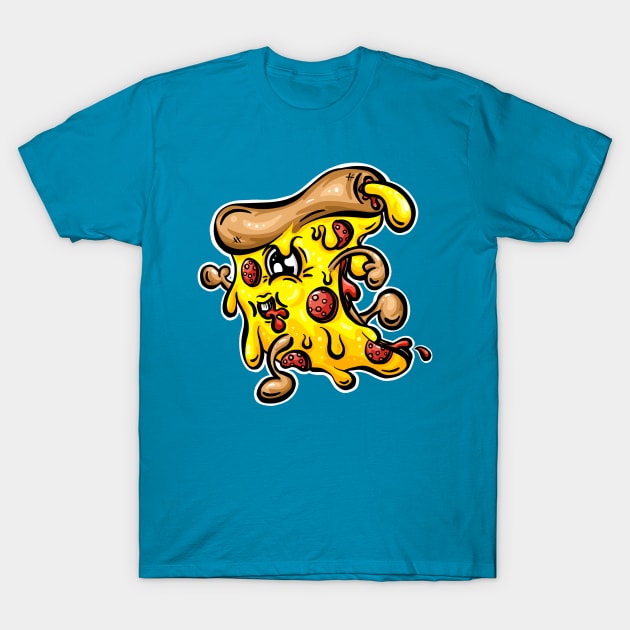The image features a teal-ish blue crew neck t-shirt laid out on a plain white background. The front of the t-shirt is adorned with a cartoon illustration of a lively, anthropomorphic slice of pepperoni pizza. The pizza slice, depicted in vibrant yellow cheese with red pepperoni spots, appears to be in mid-run from right to left, exuding a gooey, melty appearance with cheese and sauce dripping down. It has animated facial features, including one eye, a mouth, and small arms and legs made of crust, all contributing to its energetic, almost frantic demeanor. The entire design is encapsulated within a white outline, emphasizing its playful and whimsical nature.